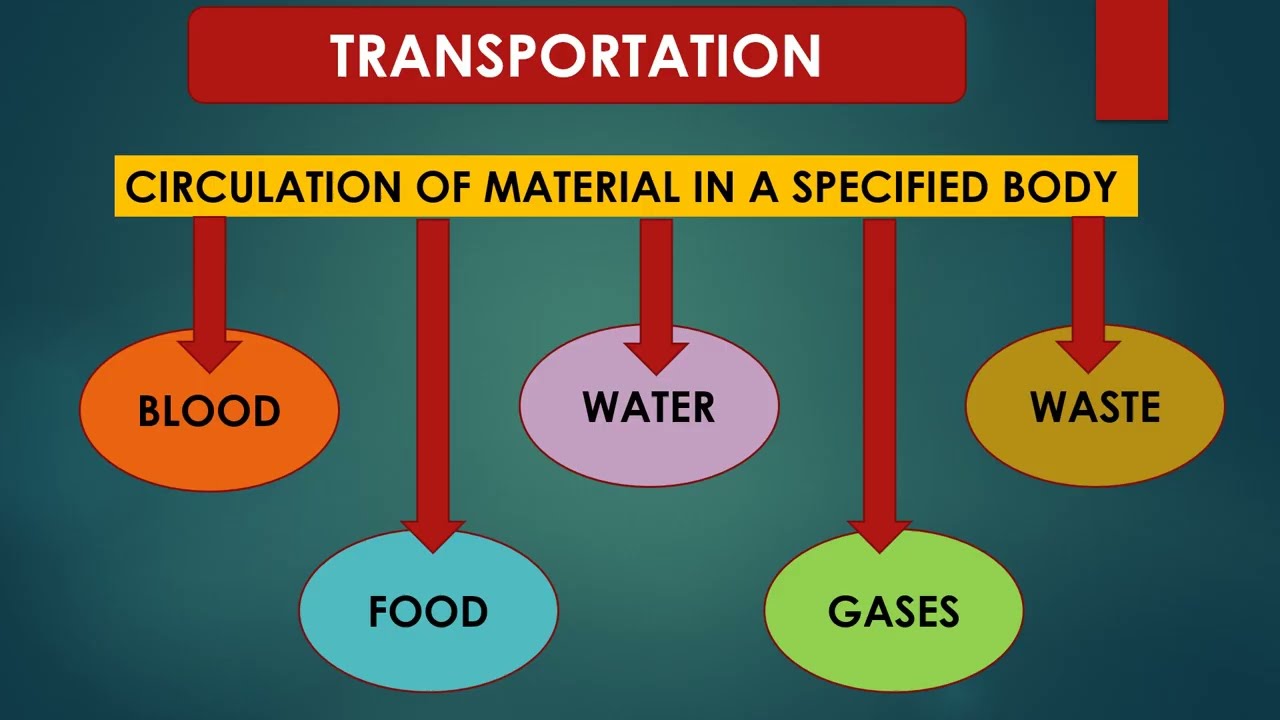The infographic features a green background with a gradient effect, the center being the lightest and darkening radially. Dominating the top edge, a red rectangle with "TRANSPORTATION" in all-caps white font is prominently displayed. Directly beneath this is a yellow rectangle with black text that says "Circulation of Material in a Specified Body." From this yellow rectangle, five red arrows point downward, each leading to distinct colored text bubbles arranged in two rows. The top row features three ovals: an orange oval that reads "Blood," a blue oval that reads "Food," and a purple oval that reads "Water." The bottom row has two ovals: a green oval labeled "Gases" and a light brown oval labeled "Waste." The detailed and organized layout with clear color distinctions aids in understanding the concept visually.